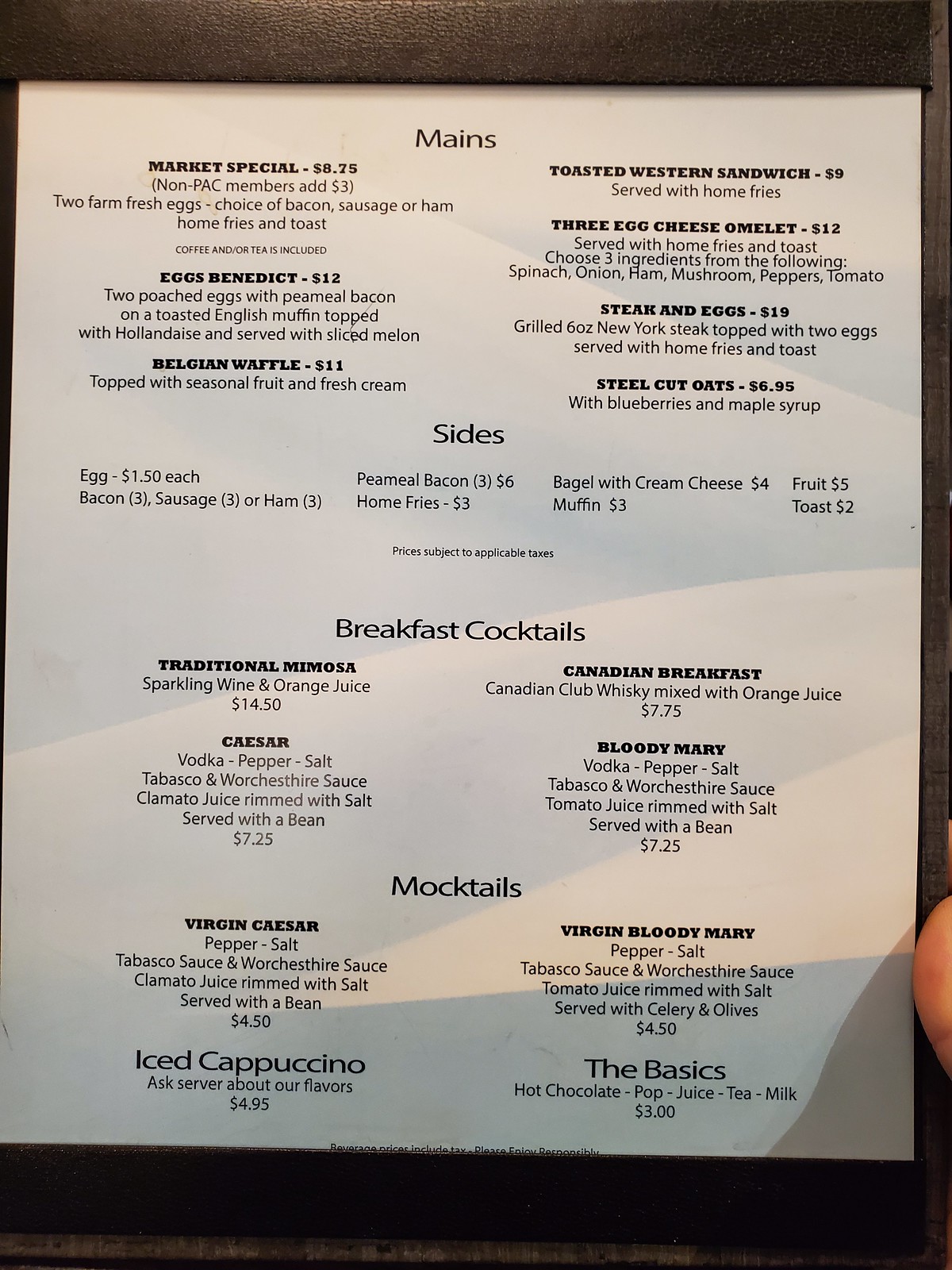A detailed caption for the described image could be:

"This image shows a white menu with black lettering, held by a person with their thumb or finger visible on the bottom right corner. At the top center of the menu, the heading 'Mains' is prominently displayed. The menu features special items such as 'Market Special Toasted Western Sandwich' on the right and 'Eggs Benedict' on the left, with 'Belgian Waffle' listed below it. To the right of the waffle, items like 'Three Egg Sandwich,' 'Three Egg Cheese Omelette,' 'Steak and Eggs,' and 'Steel Cut Oats' are detailed.

Below the 'Mains' section is the 'Sides' area, where each item is priced at $1.50 or totaling three dollars. Listed sides include sausage, pea meal bacon, home fries, bagel with cream cheese, and muffin.

Further down, the menu offers 'Breakfast Cocktails,' featuring a 'Traditional Mimosa' on the left, followed by 'Caesar,' a 'Canadian Breakfast,' and a 'Bloody Mary.' Just below, under the 'Mocktails' section, drinks like a 'Virgin Caesar,' 'Iced Cappuccino,' and 'Virgin Bloody Mary' are mentioned.

At the very bottom, under the section titled 'The Basics,' the menu includes options like hot chocolate, pop, juice, tea, and milk, each priced at $3. The menu design is straightforward, emphasizing clarity and readability with its white background and black text."